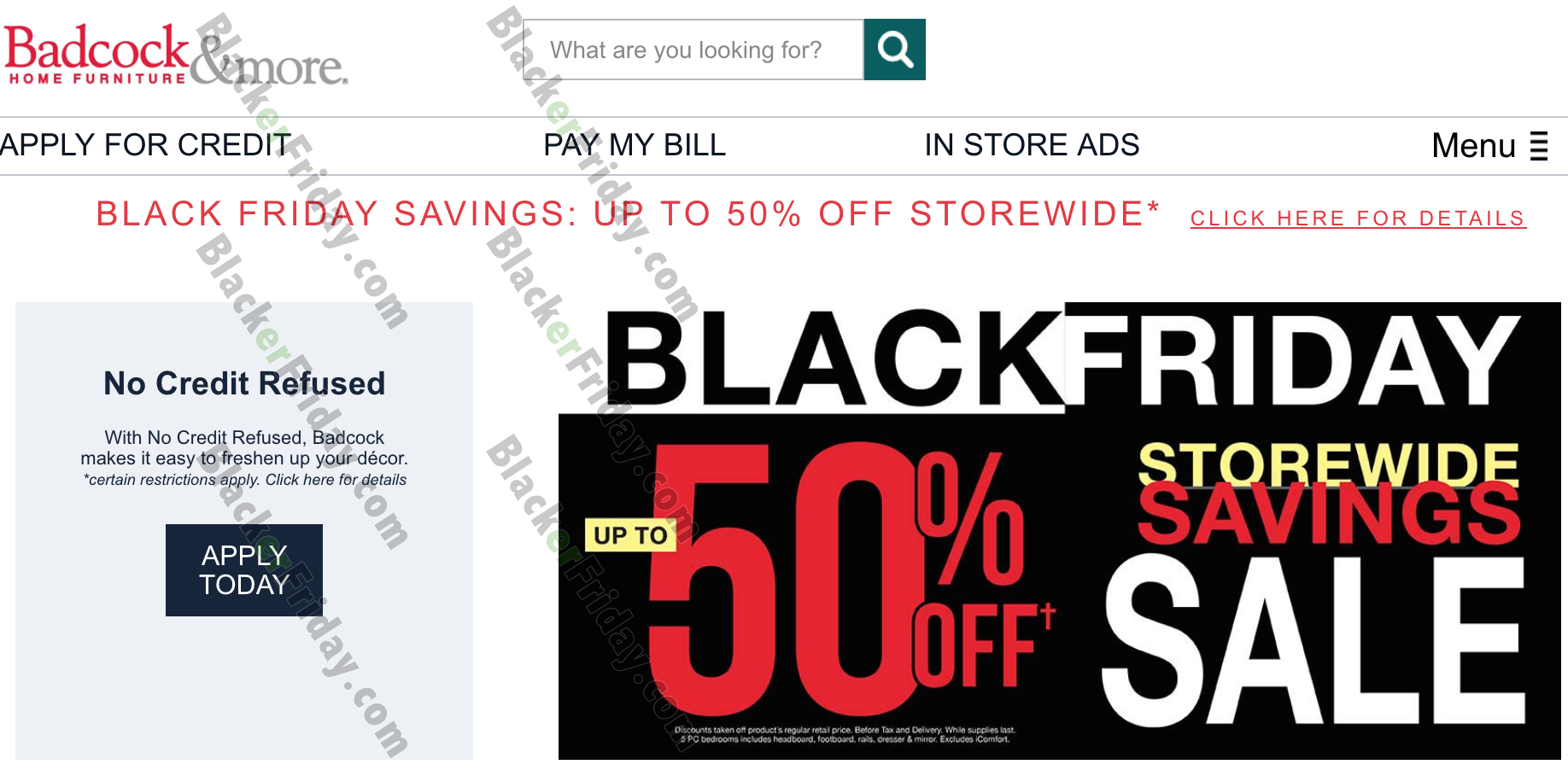Screenshot of a promotional web page for Badcock and More Home Furniture, showcasing their Black Friday deals. At the top left corner, the brand's name, "Badcock and More Home Furniture," is prominently displayed. Below it, a search bar invites users to input their queries with the text, "What are you looking for?" Adjacent to the search bar are quick access links for "Apply for Credit," "Pay My Bill," "In-Store Ads," and a "Menu."

A promotional banner near the top highlights "Black Friday Savings," announcing discounts of "up to 50% off store-wide" and encouraging users to "click here for details." Along the left side of the page, a message states, "No credit refused," emphasizing Badcock's commitment to making home decor accessible to everyone, though it notes that "certain restrictions apply" with a prompt to "click here for details."

The centerpiece of the page is a large black banner boldly declaring "Black Friday, Up to 50% Off Store Wide Savings Sale," with the fine print clarifying that discounts are applied to products' regular retail prices before tax and delivery, and are available "while supplies last." Specific details mention that five-piece bedroom sets include a headboard, footboard, rails, dresser, and mirror, though "Excludes iComfort" (with a stylized lowercase 'i' and uppercase 'C').

The left side of the image is overlaid with a watermark from "BlackerFriday.com," printed multiple times.

Note that there are no people visible in the screenshot.